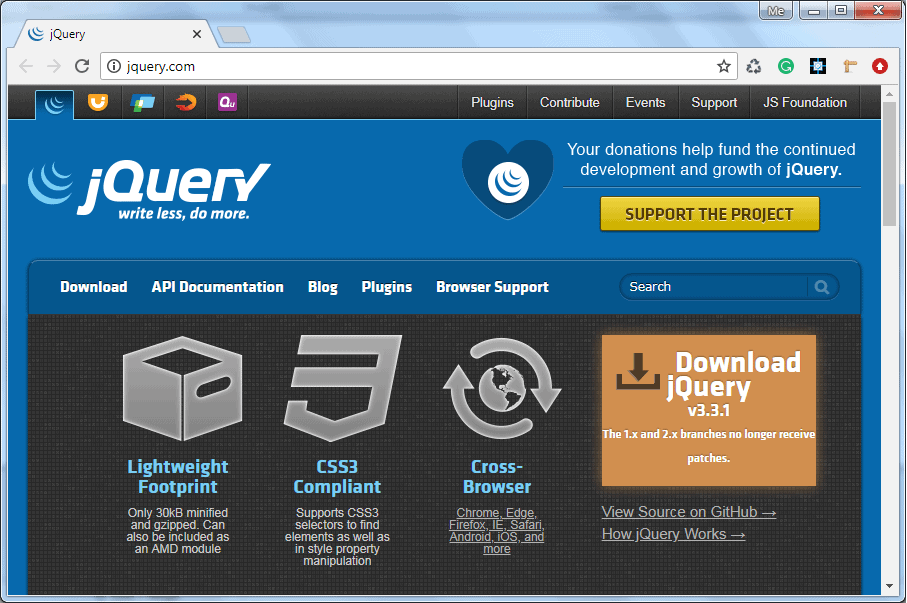"Screenshot of the jQuery Website on an Older Version of Windows"

This detailed screenshot showcases the jQuery website, viewed on an older version of the Windows operating system. The website prominently displays its name, 'jQuery,' alongside its logo, which encapsulates the slogan "Write Less, Do More." The logo is adorned with a heart and three elliptical white shapes, adding a touch of simplicity and elegance.

At the center of the screenshot, there is a clear indication that jQuery is available for download, with the current version emphasized as 3.3.1. The key attributes of jQuery are highlighted, emphasizing its lightweight nature and small footprint. It is also noted for its compliance with CSS3 standards and compatibility across multiple web browsers, including Chrome, Edge, Firefox, Internet Explorer (IE), Safari, as well as on various mobile platforms such as Android and iOS, among others.

The background of the website is rendered in a deep, dark blue, providing a sleek and professional ambiance. Most of the text is crafted in white or grey, ensuring high readability and contrast against the dark background. This attention to detail ensures that users can easily navigate and understand the essential information about jQuery at a glance.